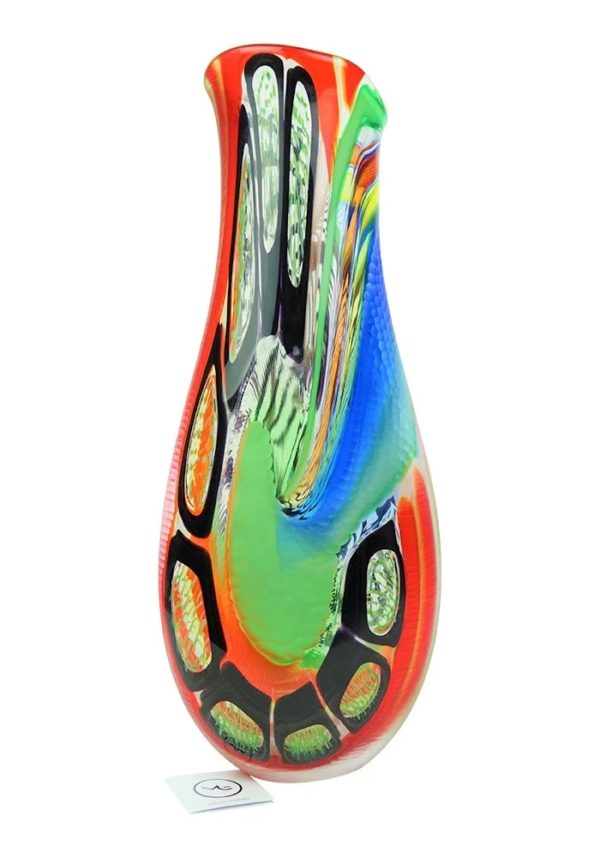This vibrant and intricate hand-worked glass vase showcases a dazzling, psychedelic mix of colors and patterns. The vase, primarily crafted from glass, features a dynamic blend of red, orange, yellow, green, blue, and black hues. Starting at the bottom, there is a swirling pattern dominated by bright red, which ascends the left side and continues onto the top lip of the vase. Embedded in this red swirl are black squares containing vivid green and orange lines, mimicking the appearance of pockets or holes. The vase also displays splashes of bright lime green in the center, which blend into blue, orange, and white streaks, creating a mesmerizing gradient and layered effect. The design includes scattered black circles and other geometric shapes, adding to its intricate and psychedelic aesthetic. The piece is angled at the top rather than being flat, giving it a distinctive and dynamic shape. Accompanying the vase is a small white card at the base, featuring a black circle with a stylized number 2 or a V logo, all set against a white background that enhances the vase's vivid colors and patterns.